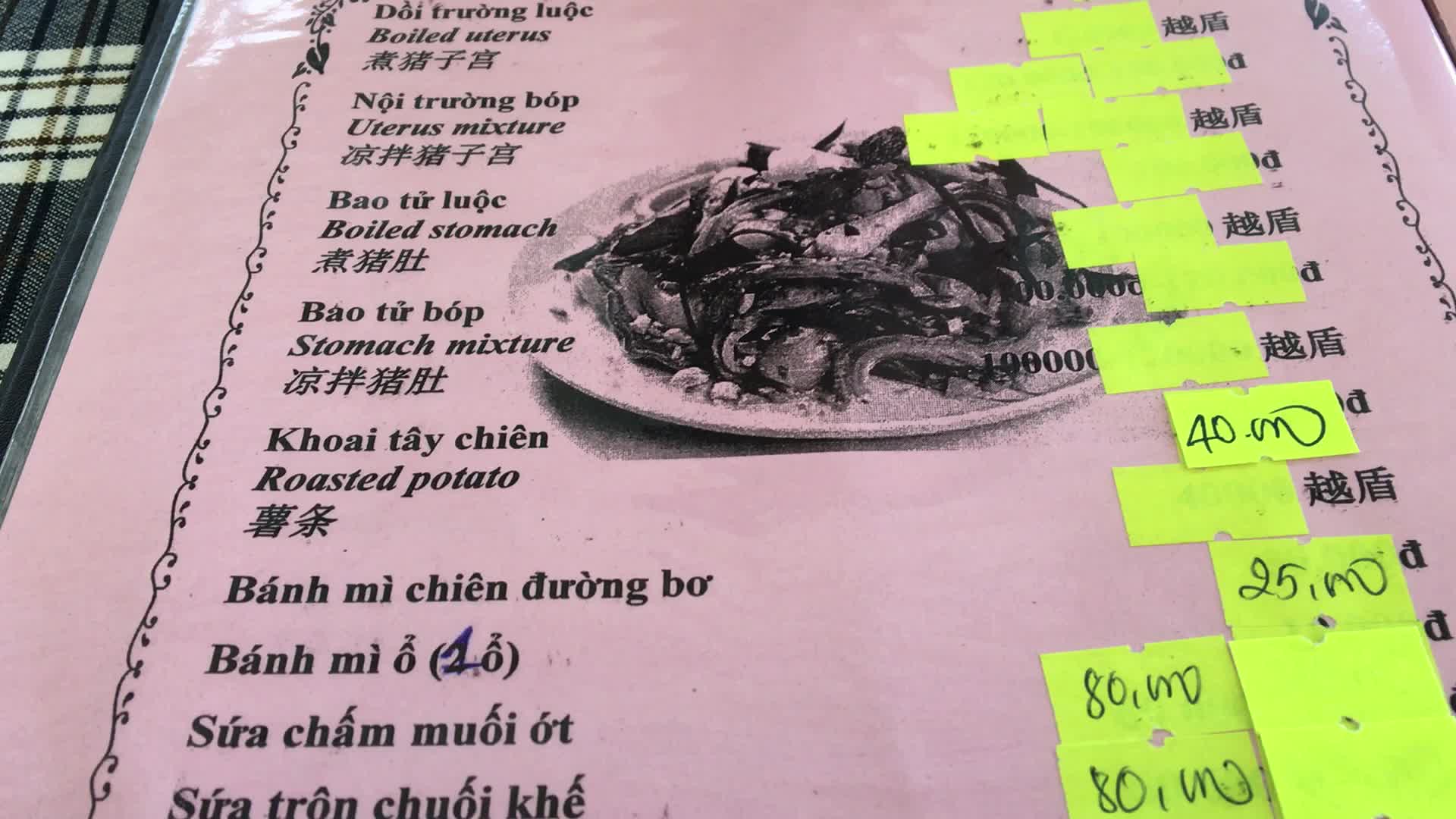The image depicts a segment of a pink menu, likely from a Vietnamese or Thai restaurant, possibly named "Bop." The pink menu is encased in plastic and lay on a gray and white tablecloth. At the center of the menu, there is a black-and-white illustration featuring a somewhat indeterminate seafood dish. The majority of the menu items have their prices and details obscured with bright yellow tape, suggesting these items may not be available. Four items, however, have updated prices handwritten next to them: 40, 25, and two instances of 80, presumably in local currency. One dish, "Surak Cham Muoi," is listed at 80 or 80,000, indicating significant alterations and age to the menu.